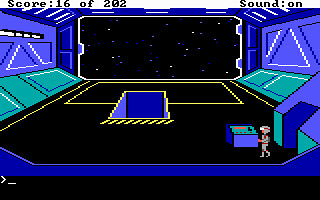This image is a screenshot from a retro-style video game reminiscent of the classic Nintendo era, evoking nostalgia similar to the pixelated charm of games like "Paperboy." The graphics are decidedly vintage, lacking modern polish and detail. At the top of the screen, in black lettering, a score is displayed: "Score: 16/202." To the right, it indicates "Sound: On." The setting appears to be the interior of a spaceship, where the walls are a blueish-purple hue, and the floor is black. A highly pixelated figure, possibly an alien or a person in a space suit, is positioned within the scene. Due to the heavy pixelation, the figure's identity is unclear. The background features a large window or screen that provides a view of outer space, depicted as a black expanse dotted with small white spots representing stars.